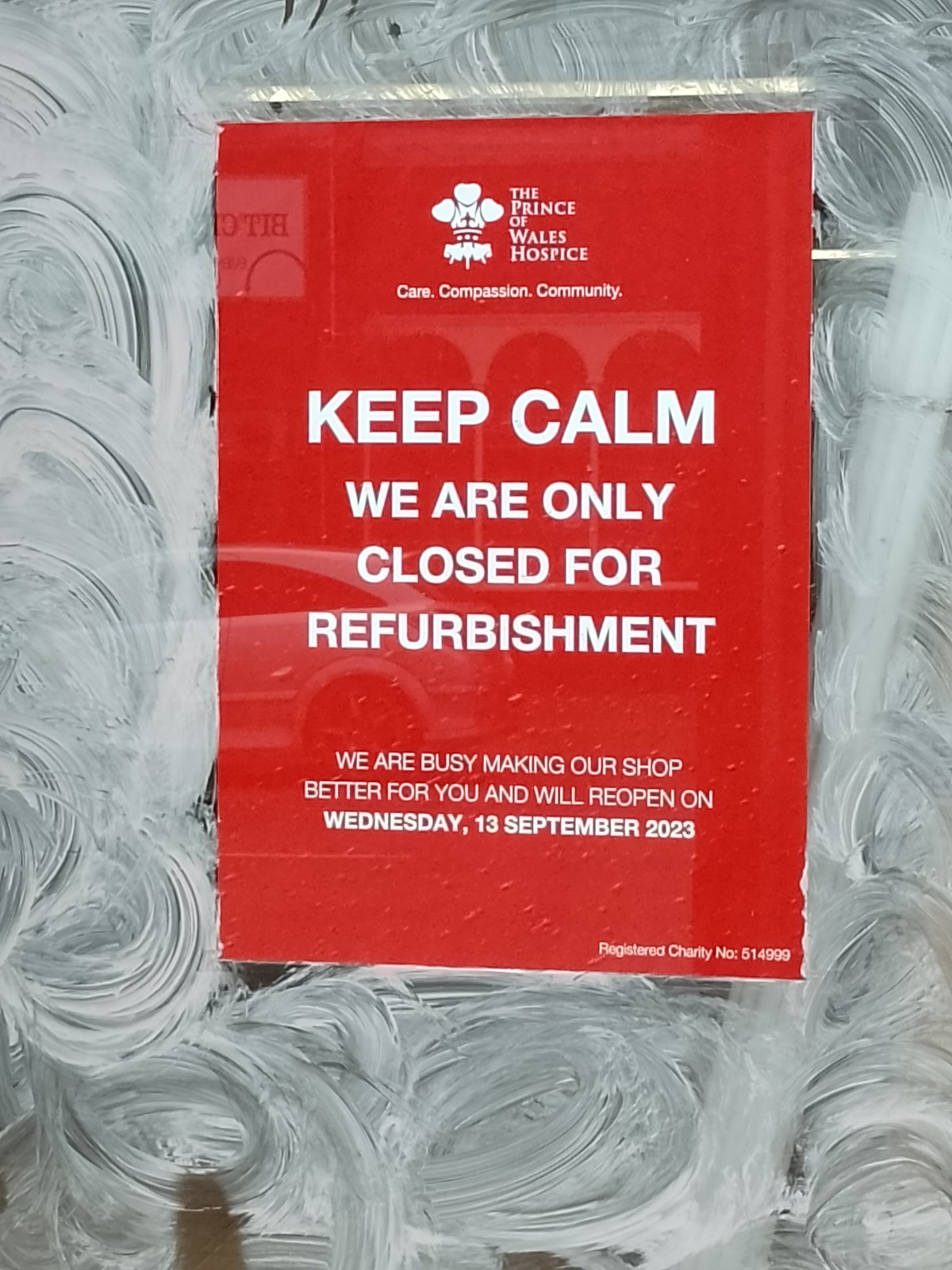The image features a red sign affixed to a smooth glass surface adorned with artistic white swirls, resembling either chalk or soap designs. The sign is emblazoned with white text of varying sizes and shapes. At the top, it showcases the logo of The Prince of Wales Hospice, which resembles a hat with a little cross and three bumps emerging from it, accompanied by the words "Care, Compassion, Community." Below this, in large, bold font, the sign reads, "KEEP CALM WE ARE ONLY CLOSED FOR REFURBISHMENT." Additional text informs viewers, "We are busy making our shop better for you and will reopen on Wednesday, 13th September 2023." In the bottom right corner, the message concludes with "Registered Charity Number 514999." The sign itself appears slightly off-center, more towards the top but almost centered both vertically and horizontally on the window.